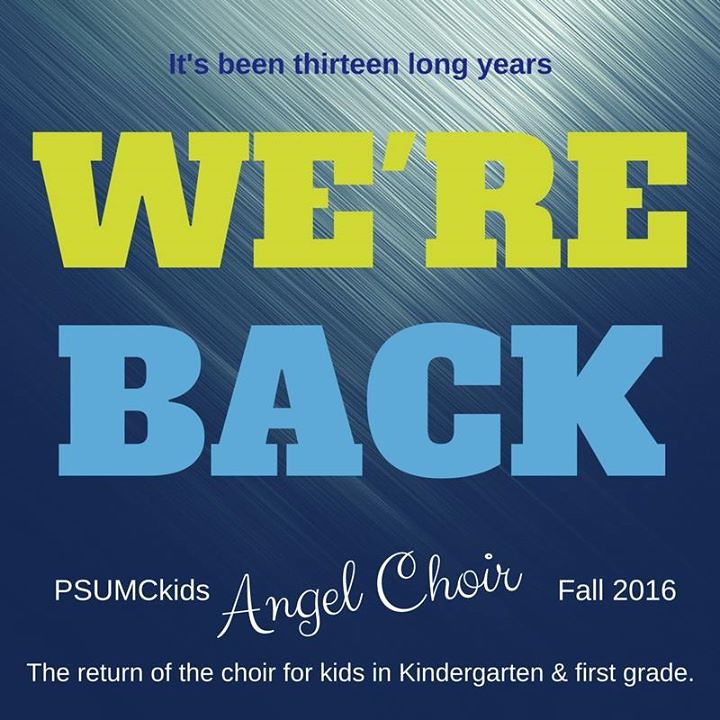The advertisement flyer features a textured, dark blue background that transitions to lighter gray tones toward the top right corner, with streaks and brush strokes adding depth and visual interest. At the top center, in small blue letters, it states, "It's been 13 long years." Below, in large, bold letters, the main highlight reads, "WE'RE" in yellow and "BACK" in blue. Further down, it announces the "PSUMC Kids Angel Choir" with "Angel Choir" elegantly written in cursive. The flyer specifies "Fall 2016" on the right. At the bottom, in smaller white letters, it proclaims, "The return of the choir for kids in Kindergarten and First Grade."